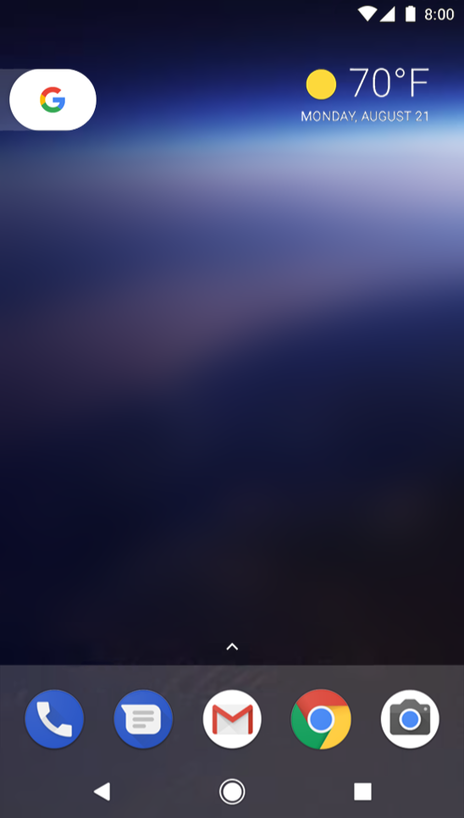This screenshot, captured from a vintage Android device, potentially a Motorola, Samsung, LG, Huawei, or another model, showcases a home screen at 8:00 AM/PM. The image suggests it was taken in a location with sunny weather at 70°F, approximately on Monday, August 21st. Prominently featured apps include Google, Gmail, a telephone app, a walking app, and a camera app, among others. The device's interface includes a central home button at the bottom for quick navigation back to the home screen. The background theme of the screen is composed of dark blue and black tones, adding to the vintage aesthetic of the device.